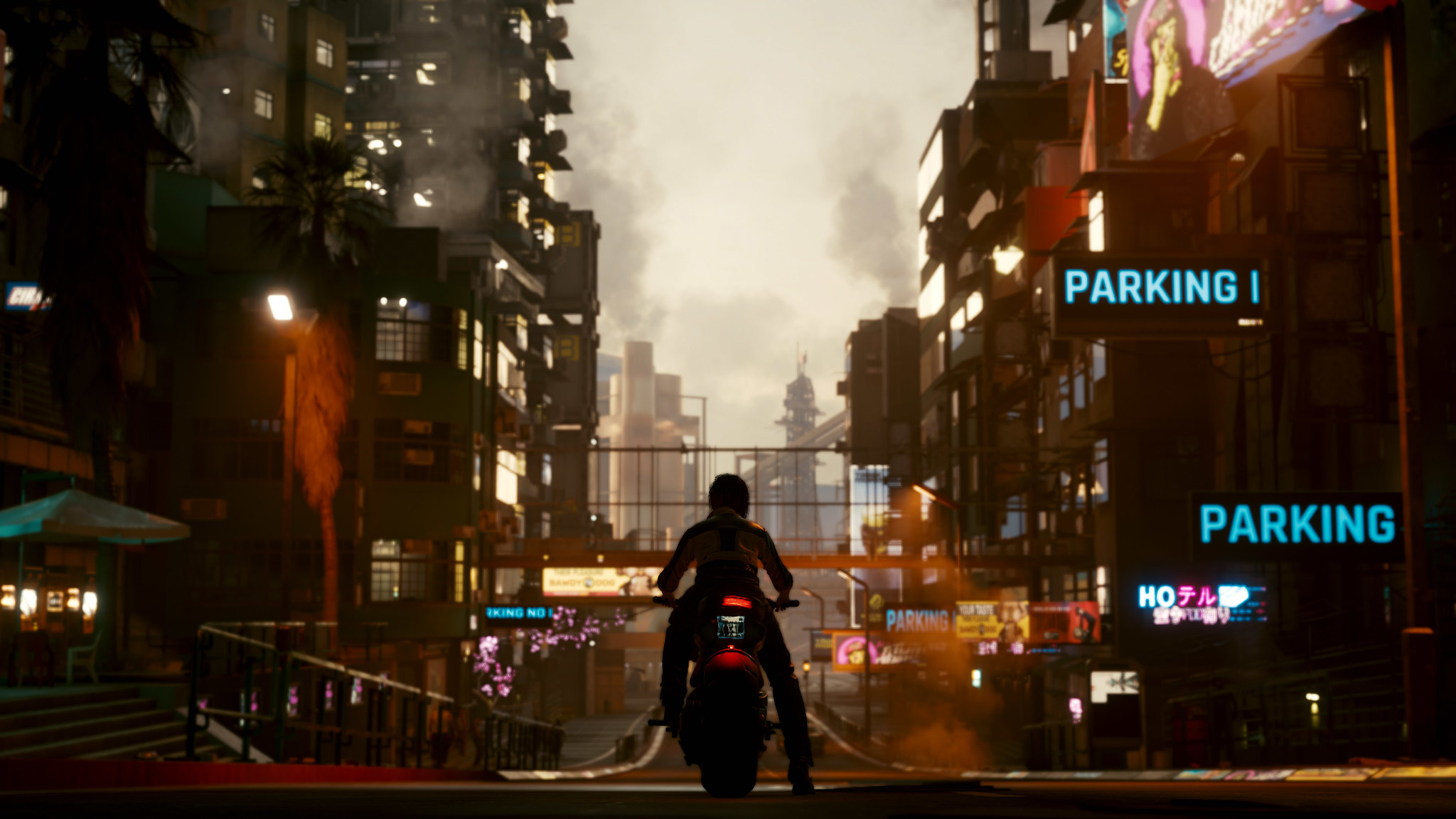A person clad in a black motorcycle suit and helmet sits astride a black motorcycle in this striking horizontal color image. The scene captures the individual from behind as they gaze down a bustling street flanked by buildings illuminated with vibrant neon signs, glowing against the twilight sky. On either side of the street, commercial establishments and apartment buildings stretch upwards, some adorned with palm trees. Scattered along the road are at least four "Parking" signs alongside others, with some displaying Japanese characters, suggesting an urban Asian setting. The image hints at a contrast between the modern glow of neon lights and the older, smokier factories in the background. Lamp posts cast shadows on the scene, while the sky in the distance remains softly lit, creating an ambiance that feels both futuristic and grounded in the present.